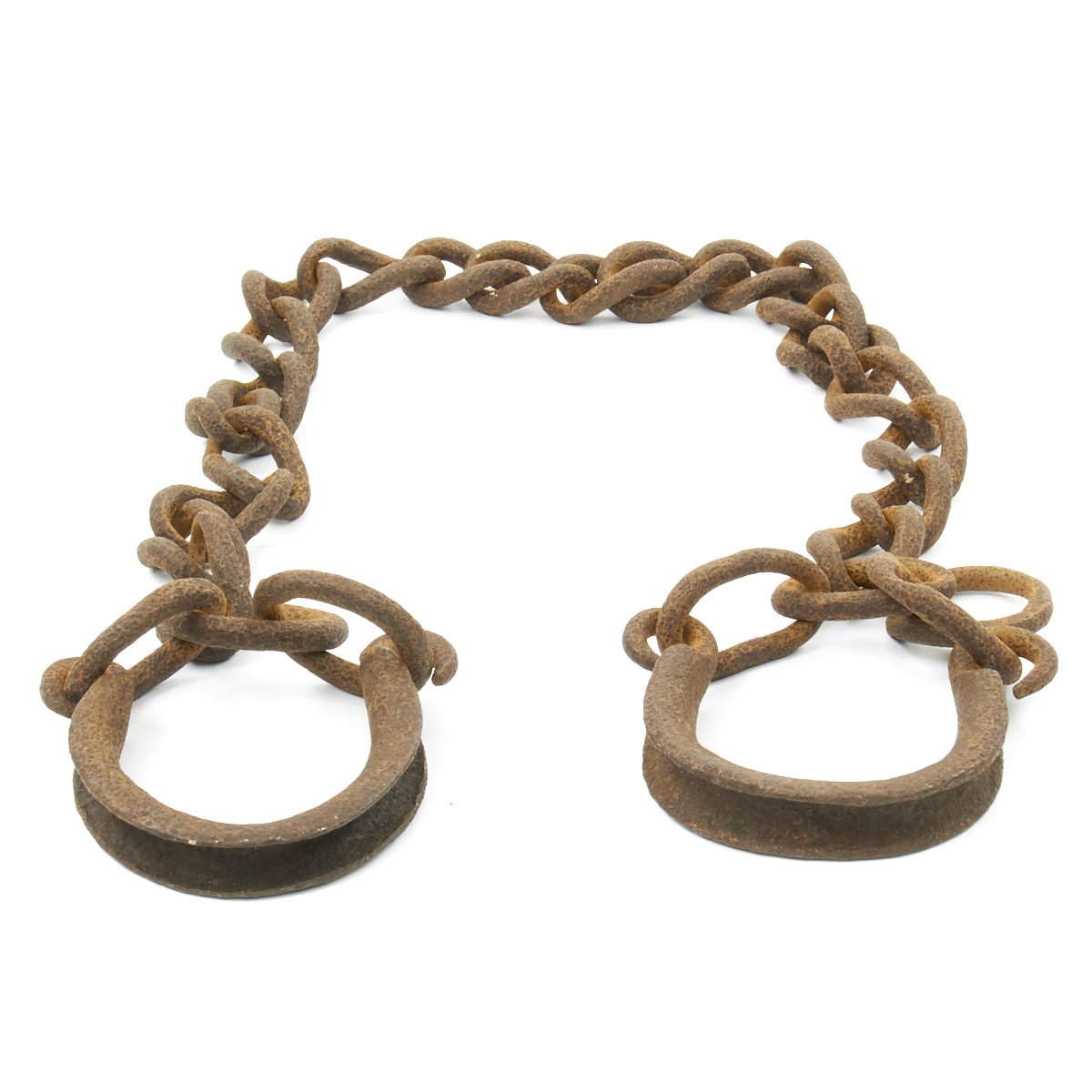This image features a pair of old, rusty metal shackles against a plain white background. The shackles have a brownish, reddish hue and exhibit significant rust, giving them an antique appearance. Designed to be worn around a person's ankles, the shackles are connected by a heavy, cumbersome chain comprised of approximately 23 thick links. The short length of the chain restricts movement, making it impossible for the wearer to take large steps. The overall layout of the shackles and chain forms a U-shape, and minor shadows can be seen around the objects, emphasizing their vintage and worn condition.